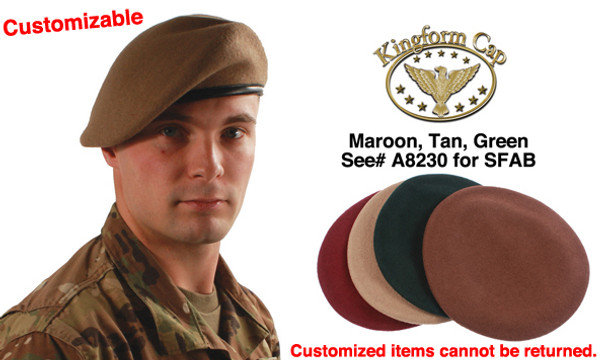This image appears to be an advertisement for a customizable military cap, set against a white background. On the left side, there is a solemn-looking soldier with blue eyes, dressed in a brown camouflage jacket over a green t-shirt, and wearing a greenish-brown beret or cap. His brown eyebrows frame a direct, serious gaze.

In the top left corner, the word "customizable" is prominently printed in red. On the upper right side, the phrase "King Form Cap" is written in gold, accompanied by an oval logo featuring a gold eagle with spread wings and surrounded by stars. Beneath the logo, black text lists the available colors: maroon, tan, green, and brown, followed by the identifier "C# A8230 for SFAB."

Below this text, an array of hats is displayed in different colors: from right to left, they are brown, black, white, and red. At the bottom of the array, a red warning states, "Customized items cannot be returned."